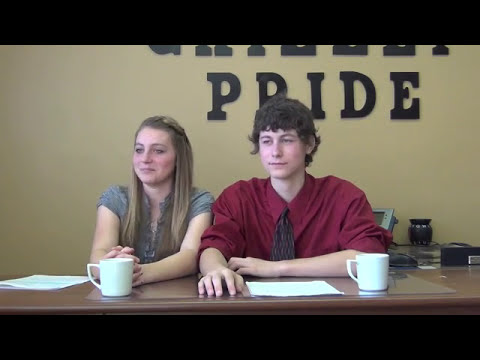The color photograph, framed with black borders at the top and bottom, depicts a man and a woman seated side-by-side at a brown wooden desk. Behind them, a beige wall features two rows of black text, with the bottom word reading "pride" while the top word is obscured. 

The man on the right has thick, short, curly brown hair and is dressed in a maroon collared shirt with a gray tie. In front of him, placed near his left elbow with the handle facing left, is a white coffee mug. His right hand rests on the desk, near a white piece of paper. The woman beside him has long, straight, blonde-brown hair and is wearing a gray short-sleeved dress. Her hands are clasped together, positioned near her own white coffee cup, which also has its handle facing left. 

Both individuals appear to be Caucasian and are looking slightly to the left with closed mouths. Additional items on the desk include multiple pieces of paper encased in a clear protective film. Behind them, there is a small black vase, a black computer mouse, and what appears to be a telephone or LED screen.